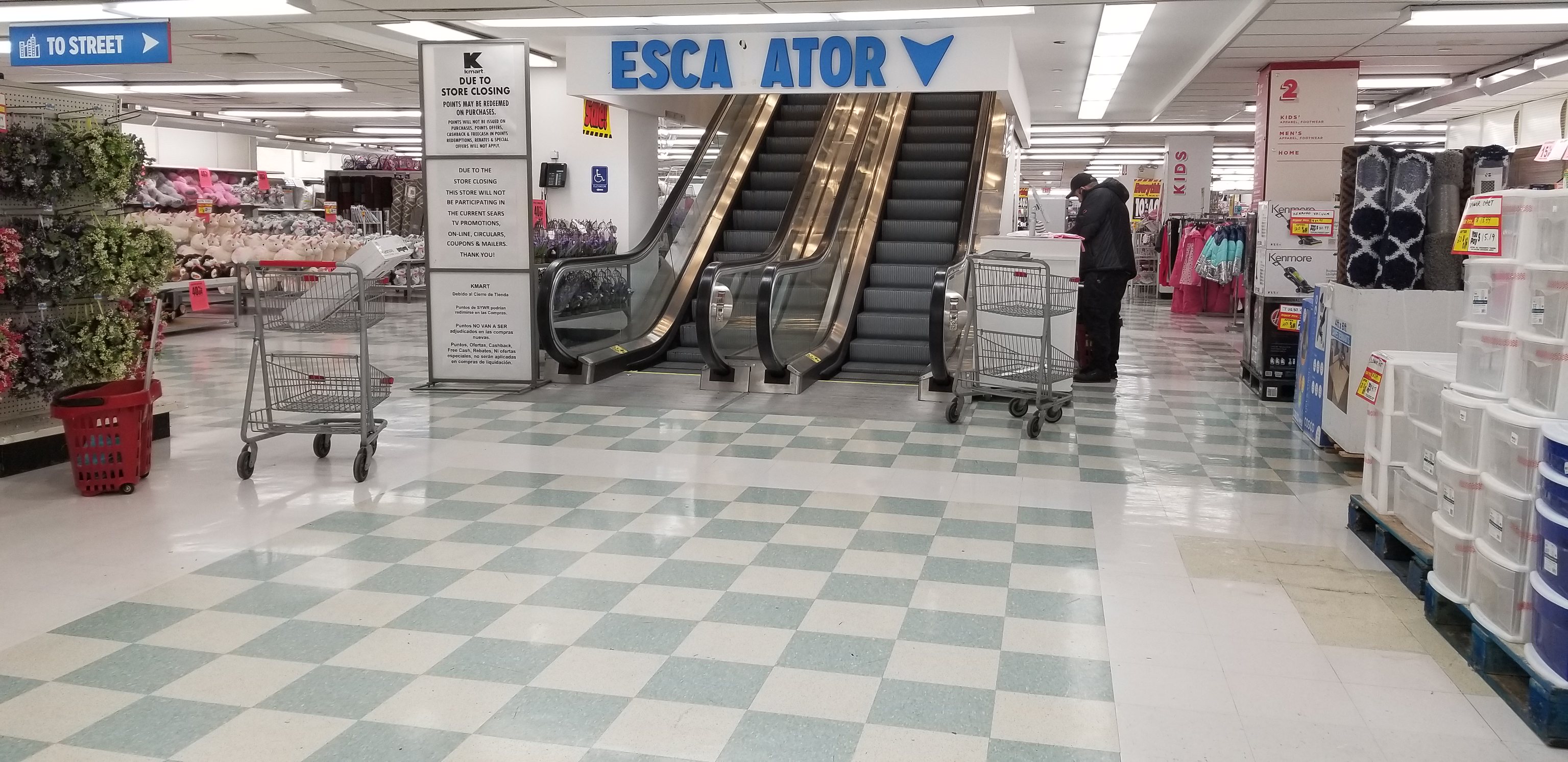The image depicts a store setting, focusing on a detailed floor pattern and various in-store elements. The floor features a central pattern of white and light bluish-gray squares arranged in vertical rows, creating an alternating checkerboard effect. To the right, there are sections of white flooring and a patch of tan square tiles. This checkered pattern continues into the distance. 

On the left, a gray shopping cart is visible from the back, next to a red shopping basket. Above these, green items are on display, and a blue sign with the text "Two Street" and an arrow pointing to the right is hung. 

The center of the image showcases an escalator with a partially missing letter in the sign above; it reads "Esca" (with the 'L' missing) and "Eder" beside a downward-pointing blue arrow. 

The right side of the image is lined with various products for sale. The ceiling is gray, featuring beams of light. There is one shopper in a black outfit, visible from a side view.